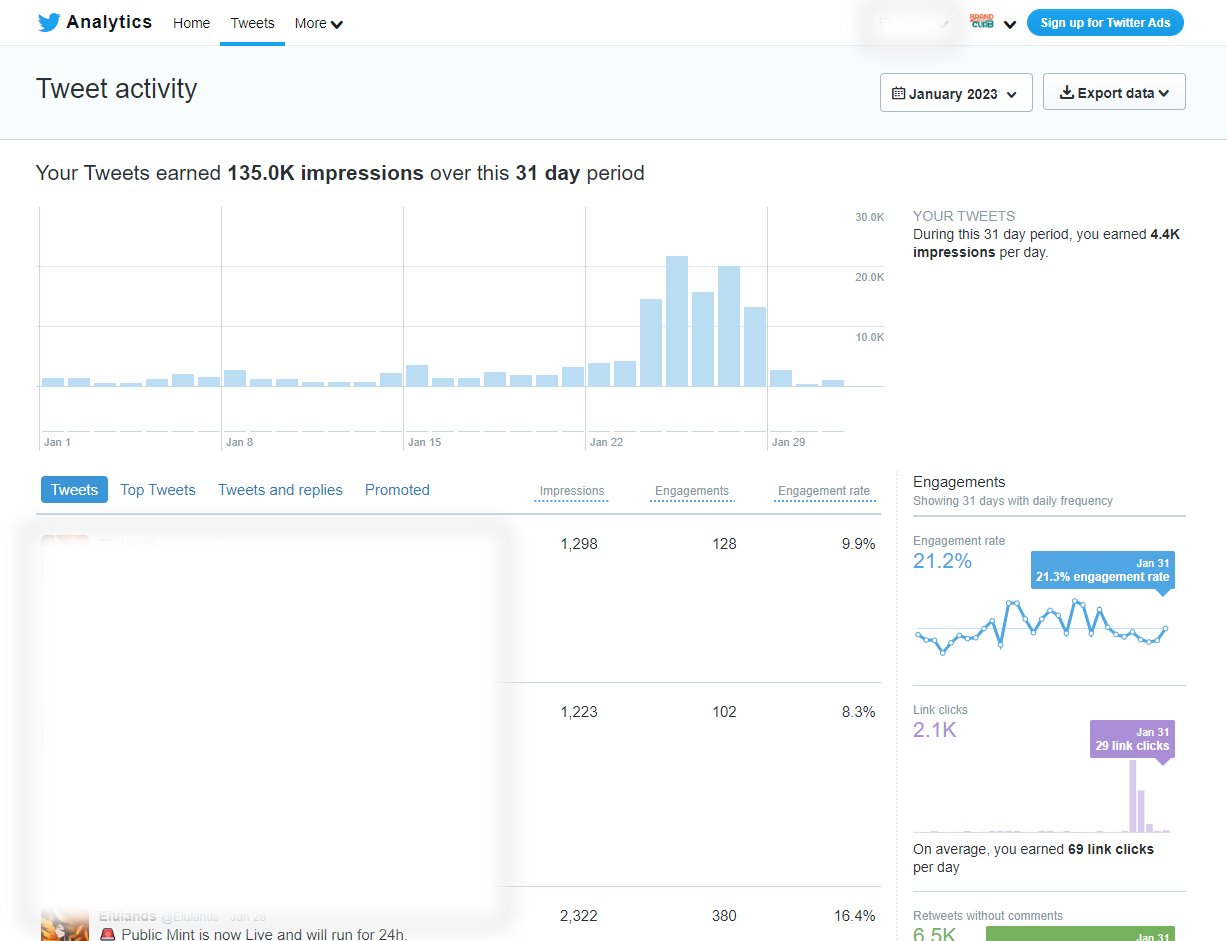Here is a detailed and cleaned-up caption for the image described:

---

The image displays the Twitter analytics dashboard for January 2023. At the very top, the familiar blue Twitter bird logo is visible, alongside navigation options labeled "Analytics," "Home," "Tweets," and "More." On the far right, a prominent blue tab invites users to "Sign up for Twitter Ads" in white text. Below that, there's a dropdown menu labeled "Brand Club," where "Brand" is highlighted in orange and "Club" in green.

Central to the dashboard is the "Tweet Activity" section, providing an overview for the entire month of January 2023. The data can be exported for further analysis. Over the 31-day period, the user's tweets accumulated a total of 135,000 impressions. 

A bar graph illustrates the daily tweet impressions, beginning on January 1st. The visual shows a fluctuating pattern with peaks and troughs throughout the month. Notably, there is a significant spike around January 22nd and 23rd, followed by a steep decline on January 29th.

Further down, specific metrics are detailed: impressions, engagement, and engagement rate. One section reports 1,298 impressions, 128 engagements, and a 9.9% engagement rate, though no specific dates are provided for this data.

To the right, another section labeled "Engagement" covers the full 31 days. It indicates an overall engagement rate of 21.2%, with link clicks totaling 2.1 thousand—an average of 69 clicks per day. Additionally, the tweets without comments garnered 6.5 thousand retweets. 

---

This detailed caption succinctly describes the key elements and data points presented in the image, ensuring clarity and coherence.